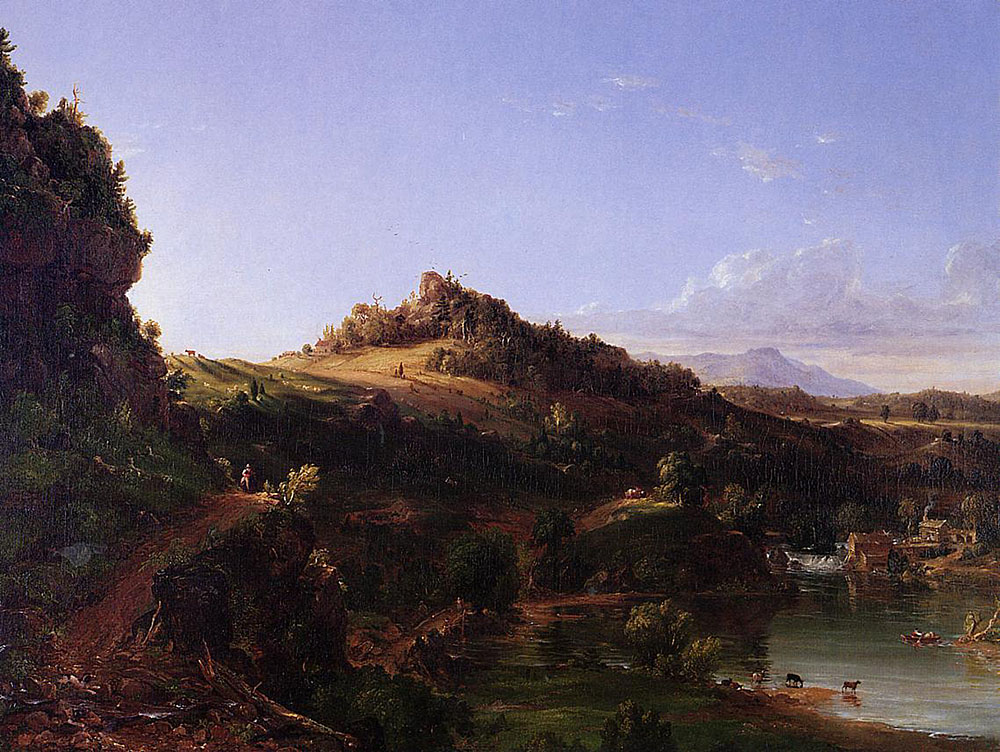This painting is a detailed landscape scene set outdoors. Dominating the background are two mountains — a prominent brown one surrounded by a vivid blue sky with heavy white clouds, and a smaller, gray mountain situated slightly farther back. In the foreground, particularly in the lower right-hand corner, a shimmering body of water can be seen with some animals, possibly cows, gathered around it, either walking or drinking from it. Nearby, across the bank of the lake, stand several buildings with gabled roofs, including an older farmhouse with smoke billowing from its chimney and men gathered nearby. A meandering dirt pathway begins in the lower left-hand corner, leading up a hill towards the distant mountains. Along this path, several small human figures are visible, dwarfed by the vastness of the natural landscape, highlighting the overwhelming scale of nature. The left side of the painting features a dense silhouette of trees, adding to the lushness of the scenery. At the hill's peak, amidst grass and dirt, more trees can be distinguished, further framing the grandeur of the scene. No text appears in this tranquil, detailed portrayal of nature's expanse against tiny human figures.